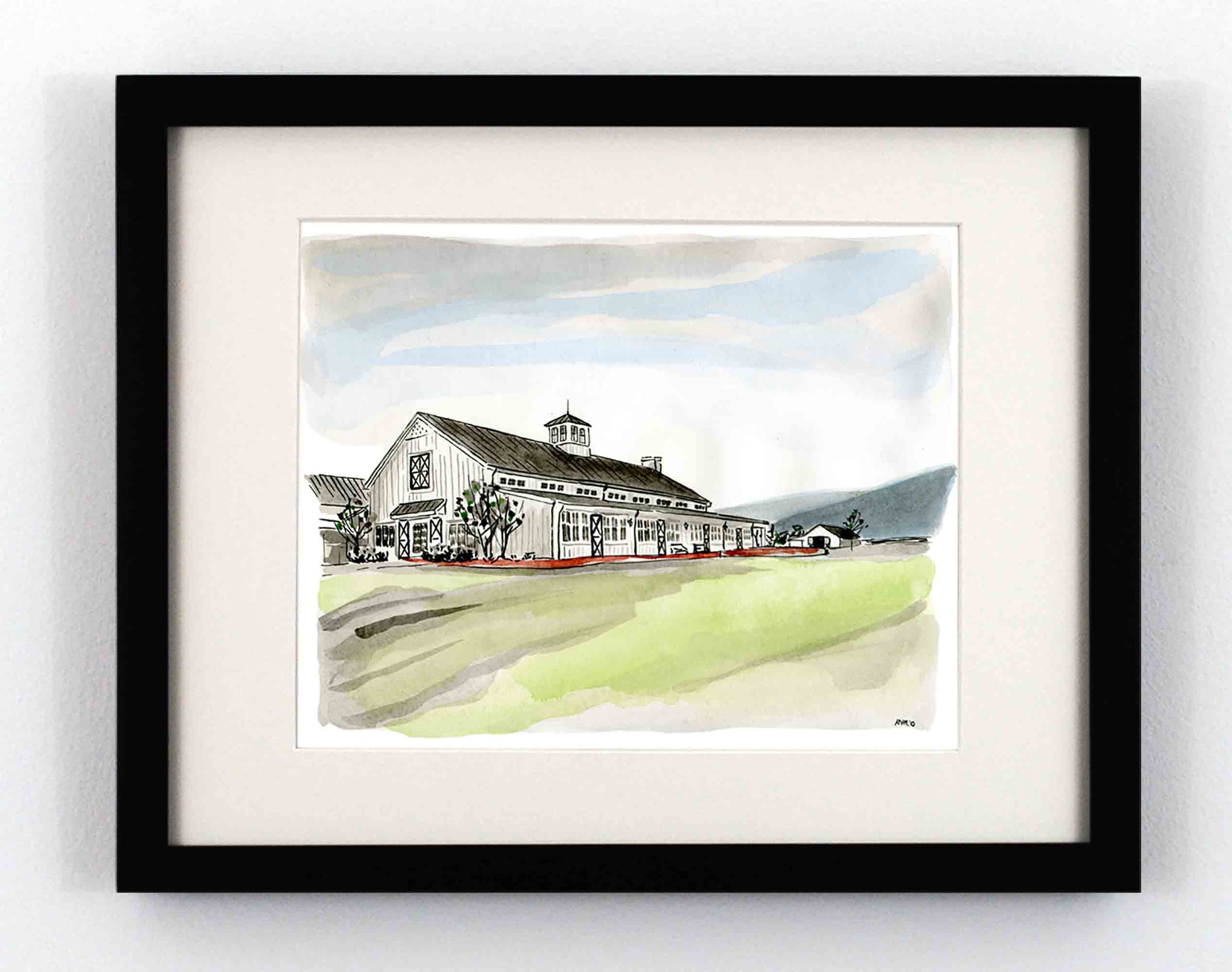The image depicts a framed watercolor painting housed in a wide, black wooden frame with a beige matte liner, surrounded by a slight white border. The painting itself features a large, old-style white house with a black roof and steeple, resembling an equestrian facility or barn. The expansive building includes several stalls or doors, each adorned with black "X" accents, and windows along each section. The front of the house features a covered porch supported by pillars, with what appears to be a small bench, and red accents suggesting parts of the porch or its outline. 

A smaller structure, also white with a black roof, appears in the background. To the left, there may be an additional wing or a garage attached to the main building. The surrounding landscape includes light and dark green grass in the foreground, with light blue sky streaked with white clouds above. In the distance, to the right, dark and light gray hills are visible. The bottom right-hand corner contains the initials "RMO" in black text. The painting is done in a realistic, photographic representational style, capturing the essence of the serene rural scene.